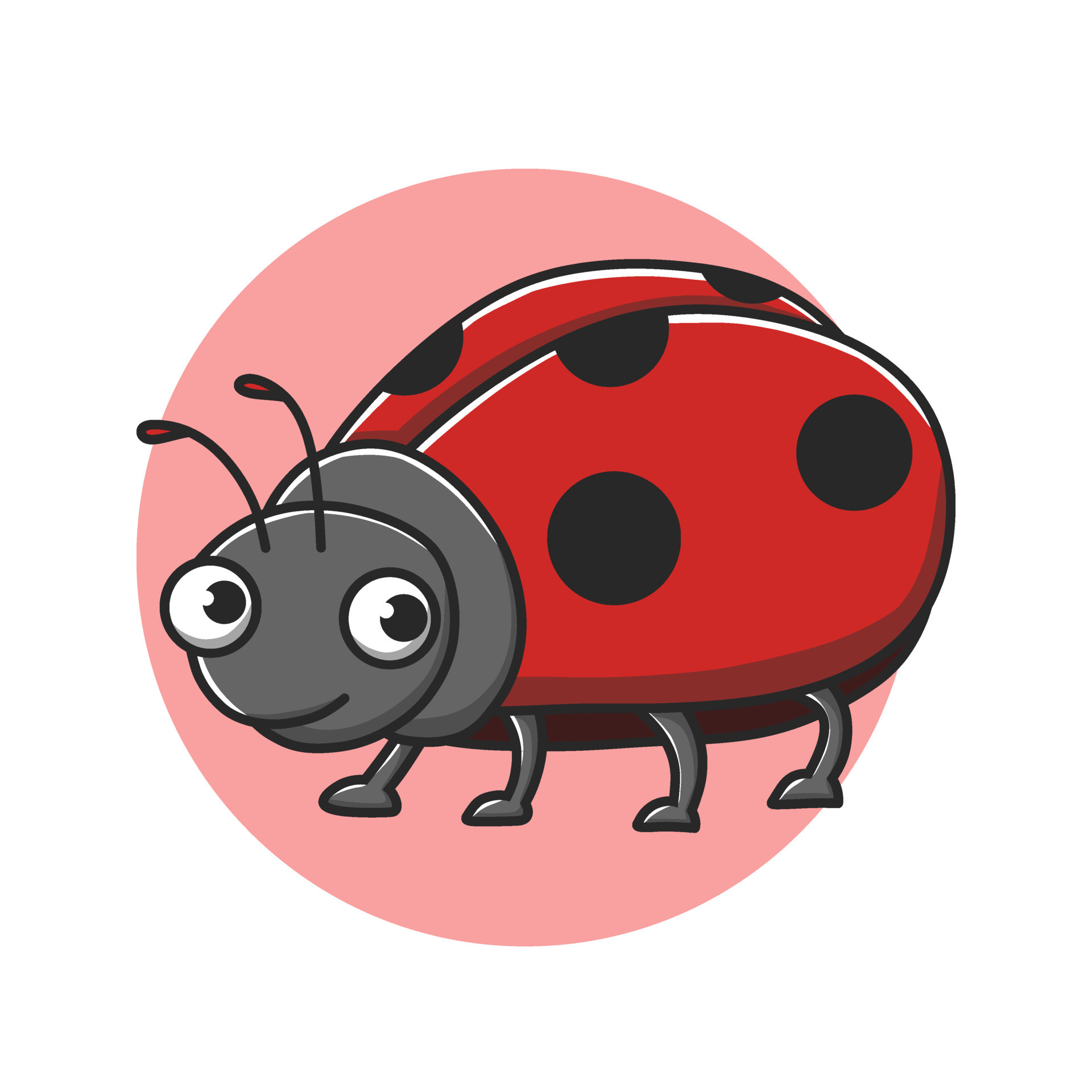This image features a cartoon-like ladybug character placed at the center of a peach-pink polka dot backdrop. The art style is simple, resembling clip art, with thick black outlines defining the shapes. The ladybug, which is facing left, has a gray head with large, googly eyes—white pupils with dark centers—giving it a cheerful and animated expression. It has a small smile and two black antennae topped with red tips. The neck area is a slightly larger gray circle. The ladybug's body consists of two oval, red wings adorned with multiple black dots, including a pair of full circles on the right-hand side and a half circle in the center. There are four thin, gray legs positioned below the body, each highlighted with white. Overall, the image exudes a playful and happy vibe, creating a charming and delightful visual.